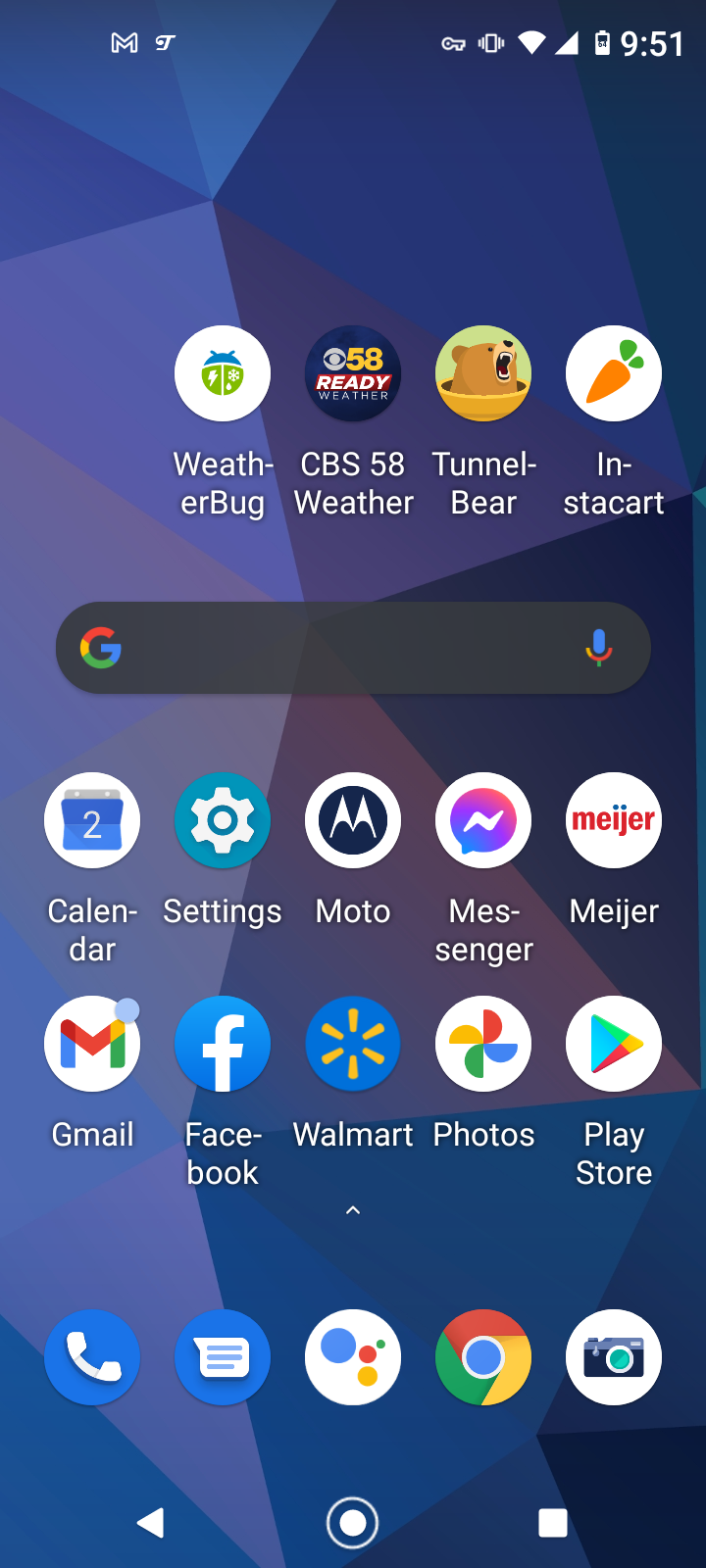This detailed description offers a cleaner and more structured caption for the image:

---

This screenshot features the home screen of a Google or Android phone, showcasing a meticulously organized layout. At the very top, the status bar displays essential icons: to the left, there is the Gmail icon and a small white icon, and to the right, the phone’s silent mode icon, Wi-Fi signal strength icon, cellular signal strength icon, battery level indicator, and the current time in the top right corner.

Below the status bar, centrally positioned, is a sleek black Google search bar. The Google logo resides on the far left of this bar while a microphone icon for voice search is on the far right. 

The background flaunts a visually appealing array of geometric shapes in various shades of blue, resembling intricate origami figures with different colored panels.

Four prominent application icons are positioned at the very top of the screen: WeatherBug, CBS 58 Weather, TunnelBear, and Instacart. Beneath these, another row features the Google search bar. 

Further below, a grid of ten more application icons is displayed: Calendar, Settings, Moto, Messenger, Meijer, Gmail, Facebook, Walmart, Photos, and Play Store.

Anchored at the very bottom of the screen is the dock, hosting the essential navigation icons: Phone, Messages, Google, Chrome, and Camera.

---

This caption captures every significant aspect of the home screen, ensuring clarity and detail for the reader.